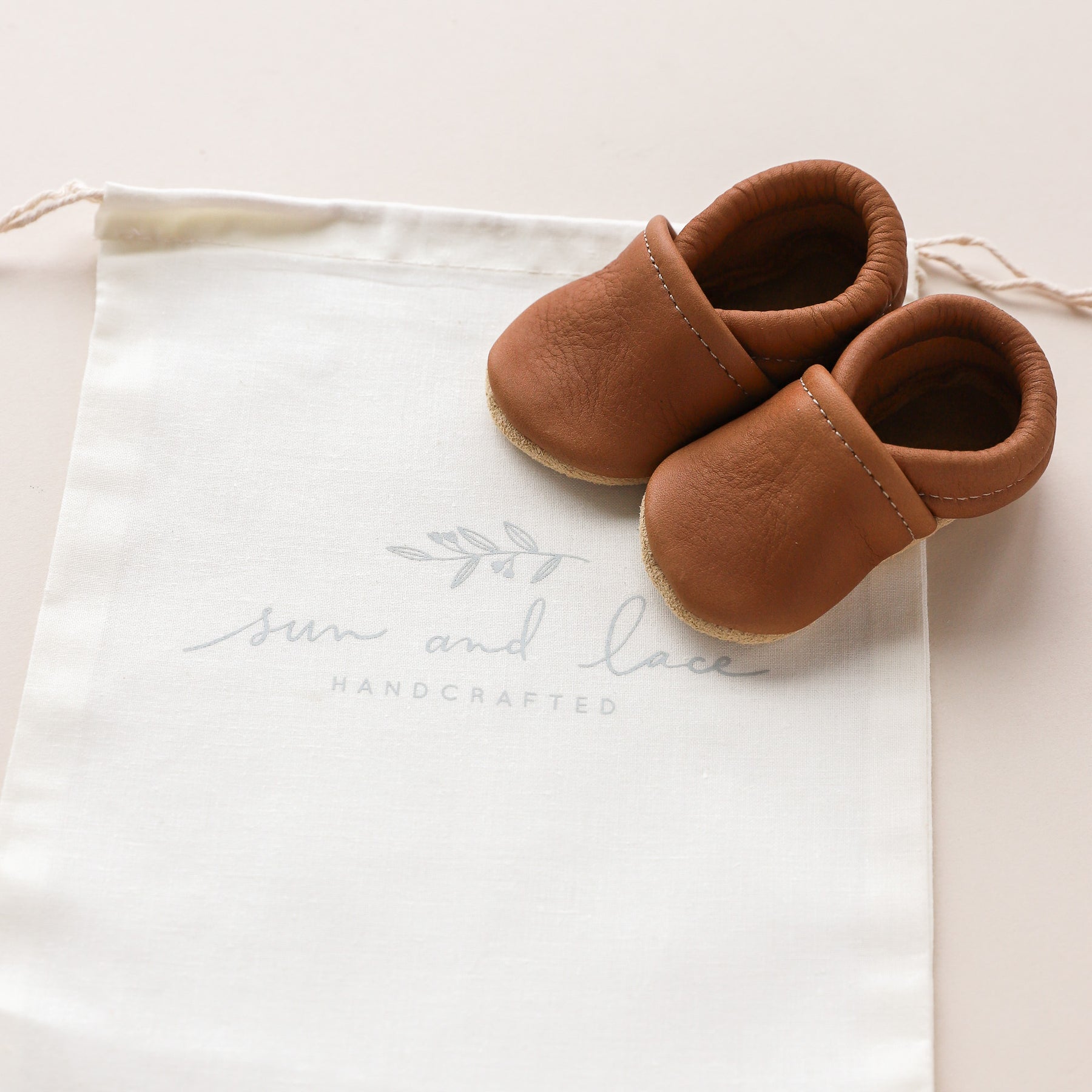The image features a pair of brown, handcrafted baby moccasins made from leather, each detailed with light tan stitching and soles that resemble cork. The moccasins are positioned diagonally, primarily occupying the upper right corner of a cream-colored drawstring cloth bag. This bag, possibly intended for storing the shoes, has delicate gray lettering that reads "Sun and Lace Handcrafted," accompanied by an illustration of a small tree branch with leaves and flowers. The entire setup rests on a light peach or tan background, highlighting the high-quality, artisanal nature of the infant footwear.